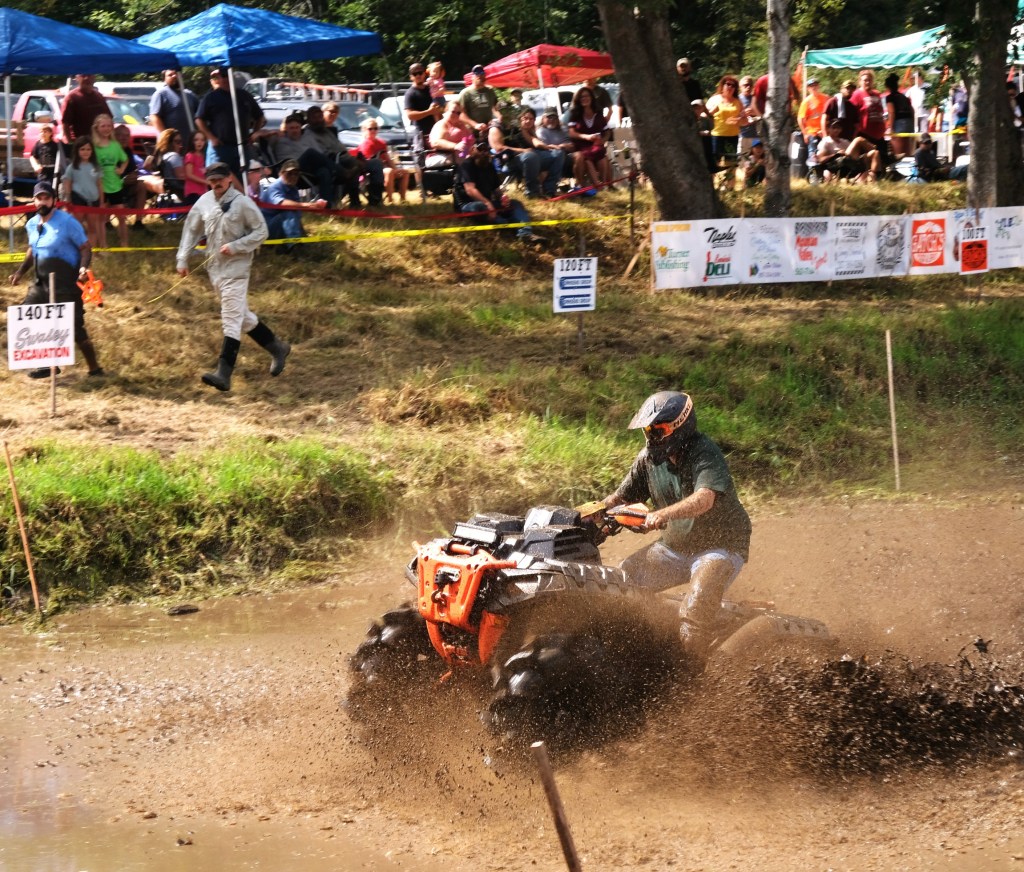The image captures a dynamic moment from an ATV derby race taking place on a muddy terrain. Central to the scene is a rider, clad in a helmet with orange goggles, a green T-shirt, and mud-splattered blue jeans, maneuvering an orange and silver ATV with enormous black tires. Mud and water spray around him, some even hitting the camera, highlighting the intensity of the race. The background features a grassy hill lined with numerous sponsor banners and signs indicating distances of 120 feet and 140 feet. Under a variety of shade awnings with blue, red, and green covers, spectators gather to watch the event. Among the crowd, a person in a white outfit and black boots is seen holding a measuring tape, collaborating with another individual in a blue shirt who is also muddy. The scene is vibrant with activity, capturing both the competition and the engagement of the onlookers and participants amidst the lively atmosphere.